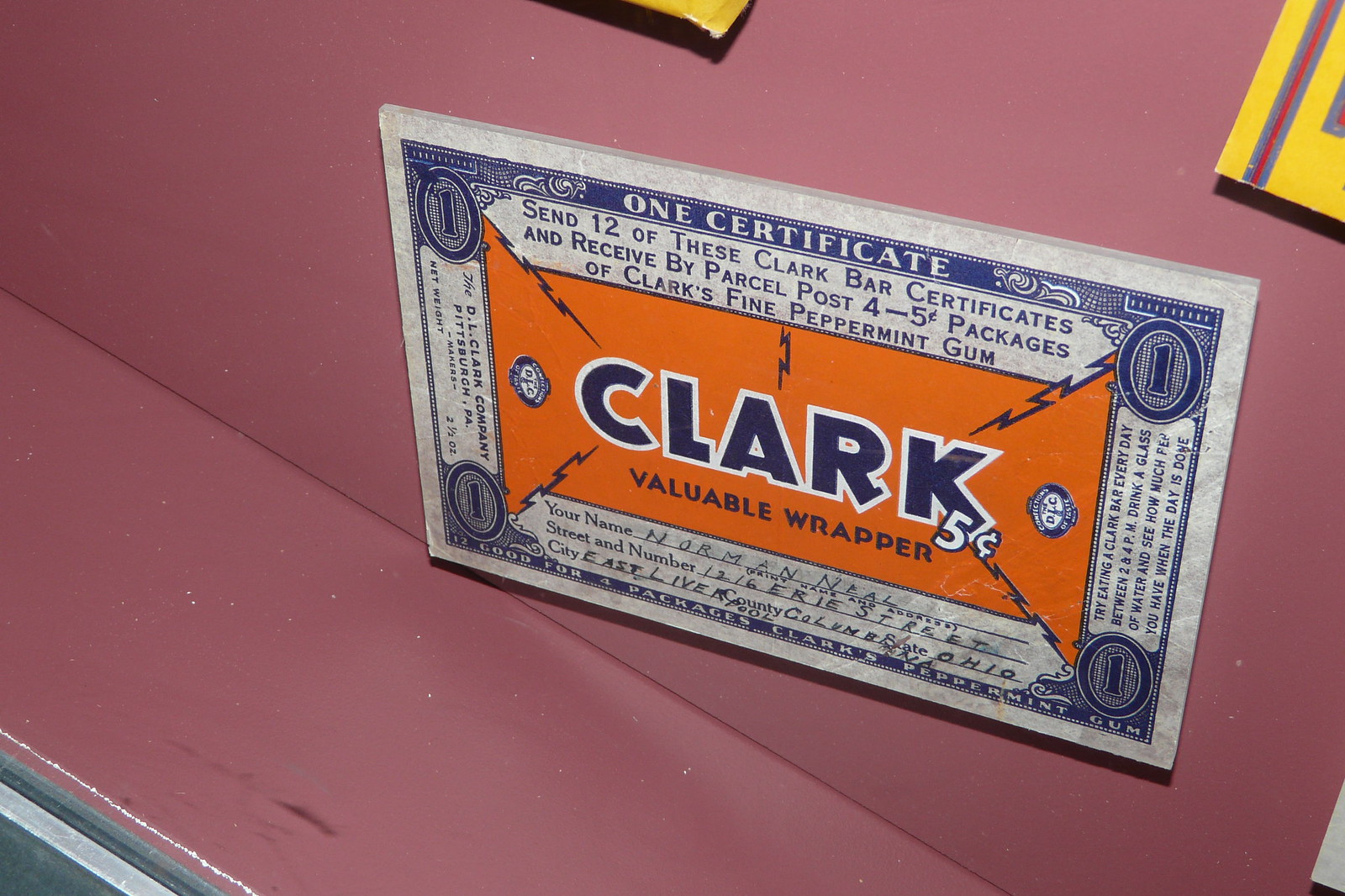The image is a detailed photograph taken indoors, showcasing a vintage gum wrapper displayed inside a tilted display case with a pink background and bottom. The display case is angled upwards from the lower right to the upper left, revealing a gray surface with white stripes along the inclined edge. Dominating the upper right half of the image is a light blue rectangle with a blue number "1" printed in a bordered rectangle at the top, labeled "one certificate." This certificate includes the following instructions: "Send 12 of these Clark bar certificates and receive by parcel post 4-5 cent packages of Clark's Fine Peppermint Gum." Beneath this, in an orange rectangle flanked by two orange triangles, the brand name "Clark" is prominently displayed in dark navy, outlined in white. The text "Valuable Wrapper" follows underneath.

At the bottom of the certificate are fields for personal information, where "Norman Neal" has handwritten his details: "26 Erie Street, East Liverpool, Columbia, Ohio." The certificate features a circled number "1" in each corner and the phrase "12 good for four packages of Clark's peppermint" along the bottom edge. The entire setup evokes a sense of early 20th-century nostalgia, highlighting the meticulous design and branding of vintage Clark's Fine Peppermint Gum.